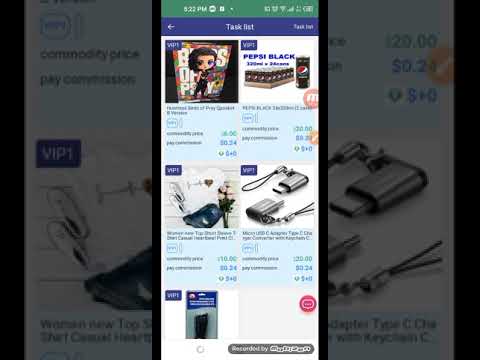The image is a screenshot, likely from a smartphone app or a webpage viewed on a smartphone. At the very top, set against a green background, are standard smartphone indicators—time showing either 8:22 p.m. or 9:22 p.m., along with battery life, Wi-Fi, and data speed icons. Beneath this is a prominent blue bar with a navigation arrow on the left, labeled "task list" centered in white text, and some unreadable text on the upper right. Below this blue bar are six panels displaying various advertisements, each with images on the top half and descriptions or prices on the bottom half. The top right panel features a case of "Pepsi Black." Other visible items include a Bratz doll, a USB storage device encased in a silver snap-together case, and a key fob. The bottom left panel, partially cut off, shows an indiscernible object with blue and white elements. The same central content is enlarged, darkened, and used as the background on the left and right sides of the image, providing a visually cohesive yet blurred border.